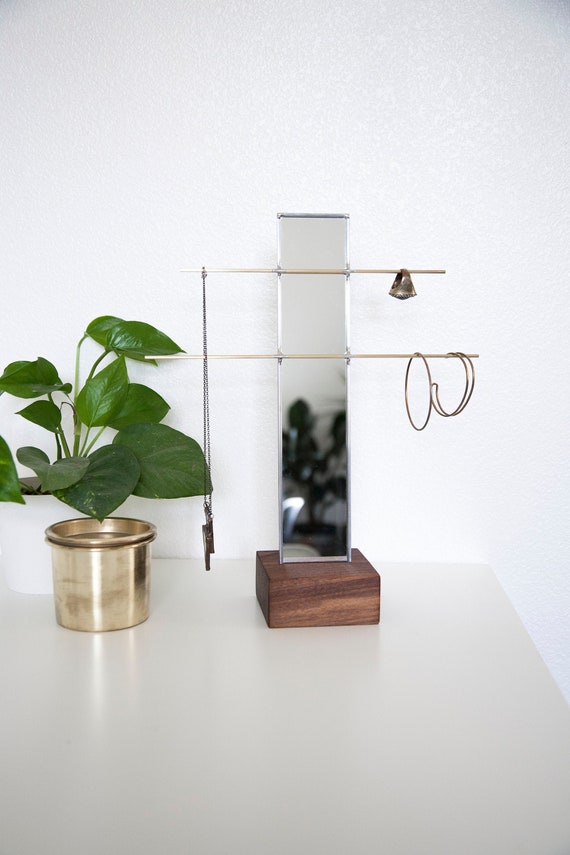A minimalist scene featuring a pristine white wall and a matching white table is showcased. On the table sits a small silver metal flower pot with a lush green plant that has vibrant leaves standing upright. Next to the pot, a unique silver metal holder is displayed, featuring two delicate arms extending outward and crowned with a small silver bell. Beneath the bell hang what appear to be two silver necklaces, adding a touch of intricate elegance. To the side, a square candle is positioned on a square block of wood. The candle has an intriguing design, with the bottom portion encapsulating a plant, while the upper part transitions into a clean white. The combination of natural and metallic elements creates a harmonious and serene aesthetic.